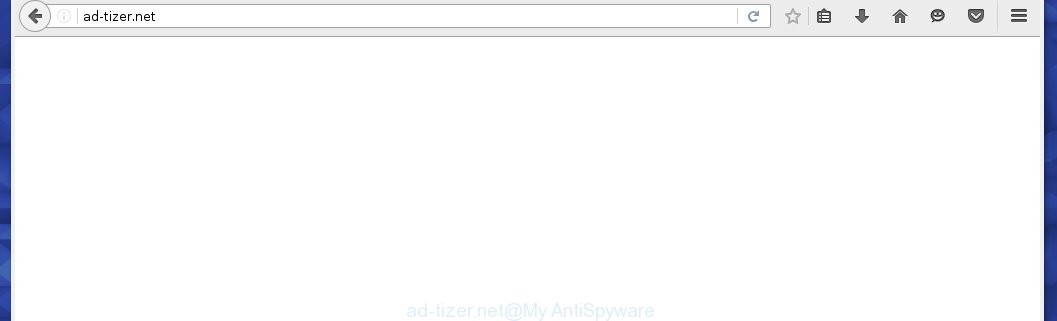The image depicts a webpage with a distinct design and layout. The borders on the left and right sides of the page are adorned with a pattern of small squares that blend light and dark blue colors, creating a visually appealing frame. The top of the page features a gray background. Within this gray section, there is a circular icon on the left side containing a black arrow pointing to the left, indicating a back function.

The address bar displays the URL "add-tizer.net". To the right of the address bar, there are several navigation and functional icons. These icons are in black, except for the refresh button and the star button, which are light gray. The icons include, from left to right: a refresh button, a star (likely for bookmarking), a trash icon, a downward-pointing arrow, a home icon, a smiley face, a shield (possibly indicating security), and a triple horizontal line icon indicating a menu or additional options.

At the bottom center of the page, light-colored text reads: "add-tizer.net at My Anti-Spyware," suggesting that the content or service might be associated with anti-spyware measures.